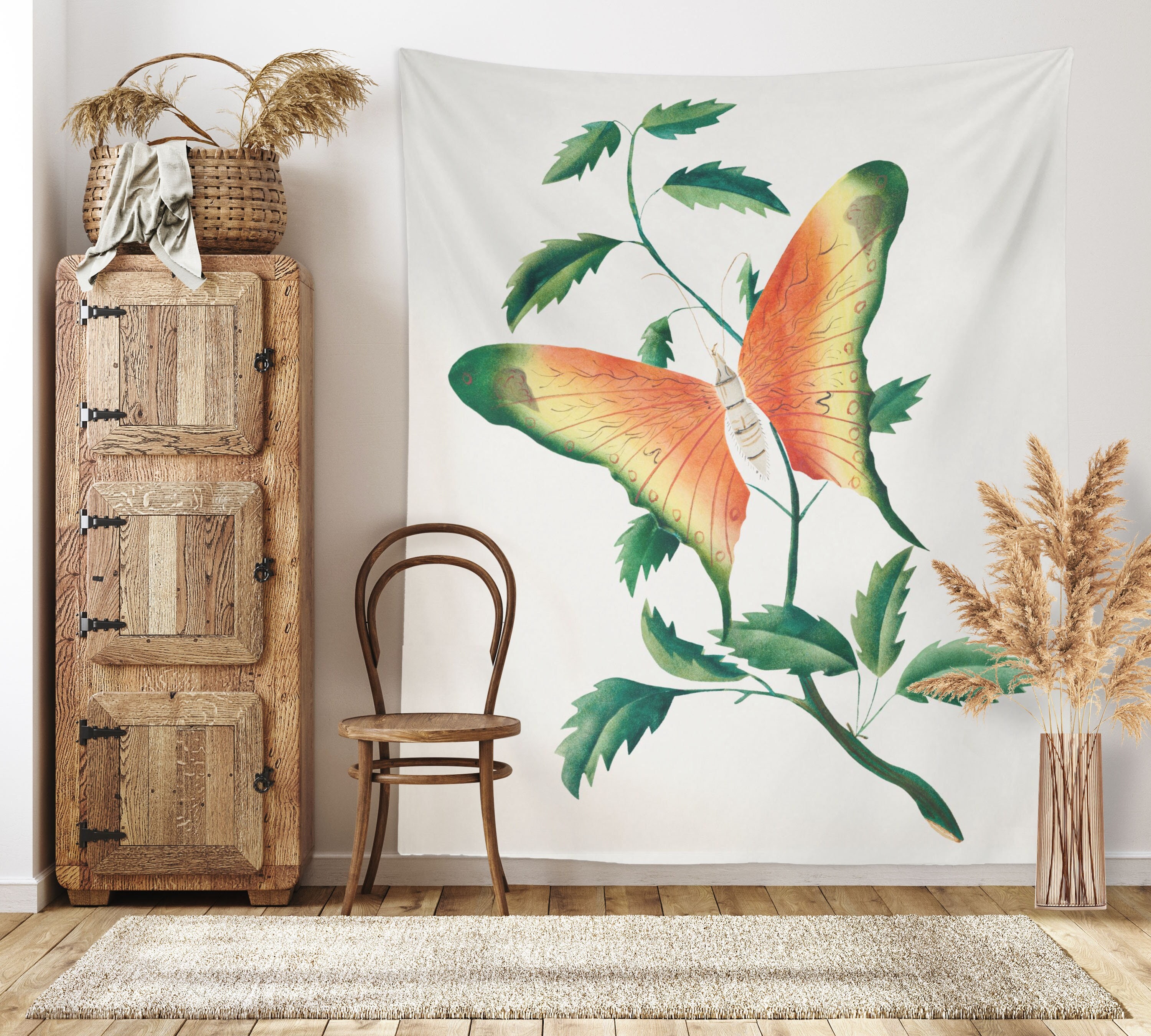This photograph captures the interior of a room with a cozy and artistic atmosphere. Dominating the wall is a tapestry featuring a vibrant mural of a large vine with a green, red, and orange butterfly hovering above it. Below the tapestry, a simple wooden chair with minimal back support sits adjacent to a vase filled with decorative, brown feathery plants that have a dried, rustic look. Covering the floor is a scratchy-looking rug in a creamish color, possibly stretching from one side of the image to the other, set against a polished hardwood floor. To the left of the chair is a wooden cabinet with three square compartment doors, each secured with black latches. On top of the cabinet is a woven basket containing what appears to be weeds and some sort of cloth. The overall composition and elements of the room radiate a calming and quaint aesthetic.